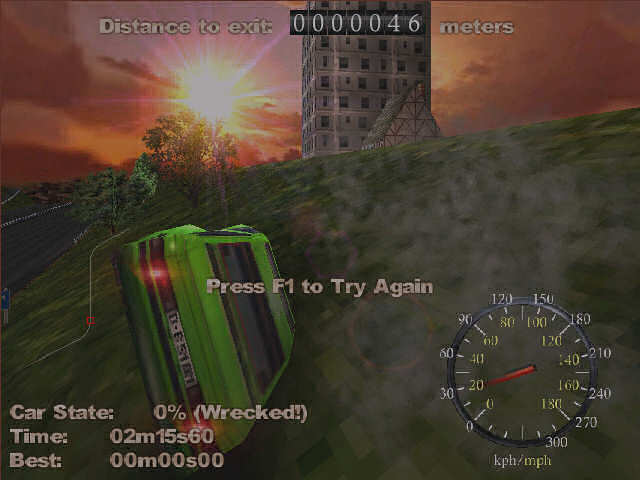This image is a screenshot from a computer game. In the foreground, slightly left of center, there is a green car that appears to be tilted onto its passenger side. The car features distinguishable red taillights and black windows. Towards the bottom right of the screen, a speedometer is visible. It is a gray circular gauge displaying white and yellow numbers, with a red needle indicating the speed. In the lower left-hand corner of the image, there is white text, though its content is not specified.

The background of the image transitions into a vibrant sky adorned with shades of orange, pink, and yellow. On the left side, the sun is depicted as a white, intensely bright circle with yellow rays emanating from it. To the right of this radiant sun stands a tall, gray square building, characterized by black windows. This building is perched on a verdant hill interspersed with patches of dirt, further enriching the scene.